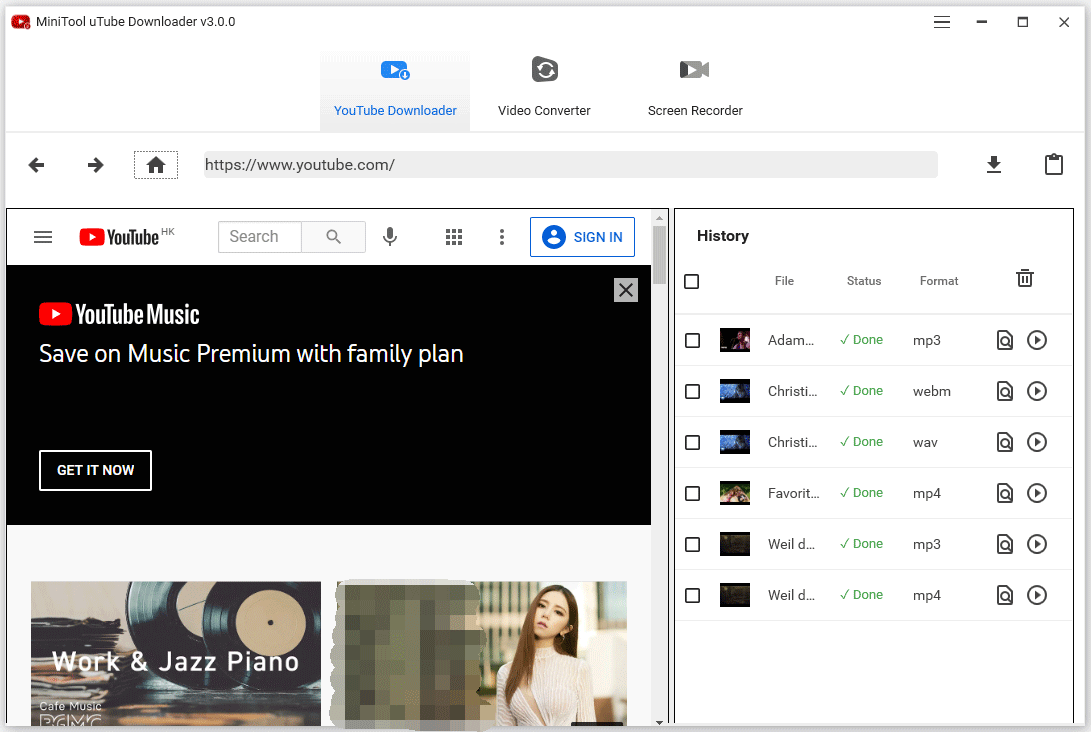A woman dressed in a white shirt sits at a piano, deeply focused on playing a jazz piece. The scene is accentuated by the presence of various digital interface elements, hinting at the multi-layered world of online music. Icons and text like "YouTube Music," "Save on Premium with Family Plan," and "Search Play" accompany the image, alongside a list of media formats such as "MP3," "WAV," and "MP4." The interface also displays options for downloading, recording, and converting videos, with tools like "MiniTool YouTube Downloader v3.0.0" clearly visible. In the background, remnants of web navigation are evident, including a back arrow, forward arrow, and URL bar, suggesting active engagement with music-related tasks. The image subtly infers the convenience and technological integration available to music enthusiasts today.